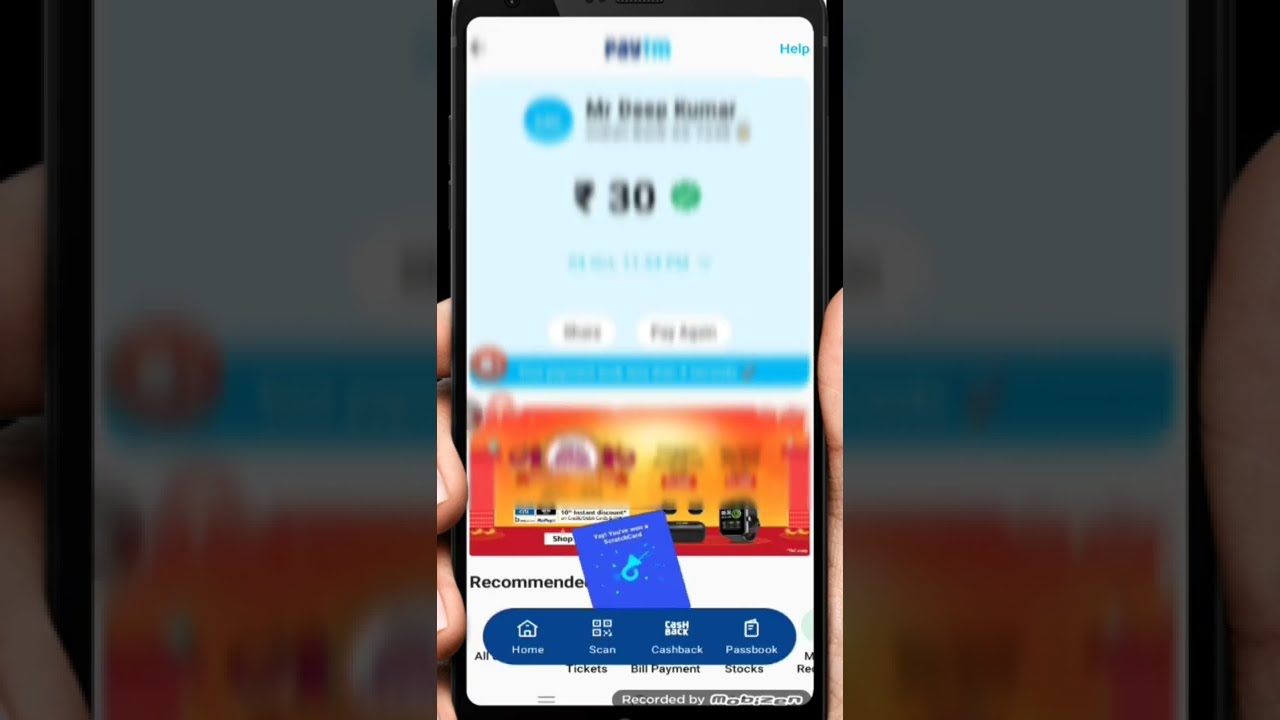The image showcases a person, identified by their barely visible Caucasian fingers, holding a cell phone indoors or possibly in a car. The central focus of the image is a somewhat blurry screen displaying a site or application. At the top in navy blue letters is the fragmented word "PAYTIN" or possibly "PAY", followed by "IM" in lighter blue. Below this, black text might spell out "Mr. Deep Rumor" or variants like "Mr. Boss Coomer". Prominently featured is the number 30 in blue.

Towards the bottom part of the phone screen, the visibility improves, revealing an orange rectangle filled with yellow and some numbers. A black line beneath this features the word "Recommended," and beneath that, blue oval icons labeled HOME, SCAN, CASHBACK, and PASSBOOK or PASSPORT in white letters. Additional text includes "TICKETS," "BILL PAYMENTS," and "STOCKS" in black, along with "RECORDED BY MOBISION" in white on a grey background.

Surrounding this central image, the entire photo's left and right thirds display an enlarged, grayed-out, and less visible version of the same scene, emphasizing the focused central portion.